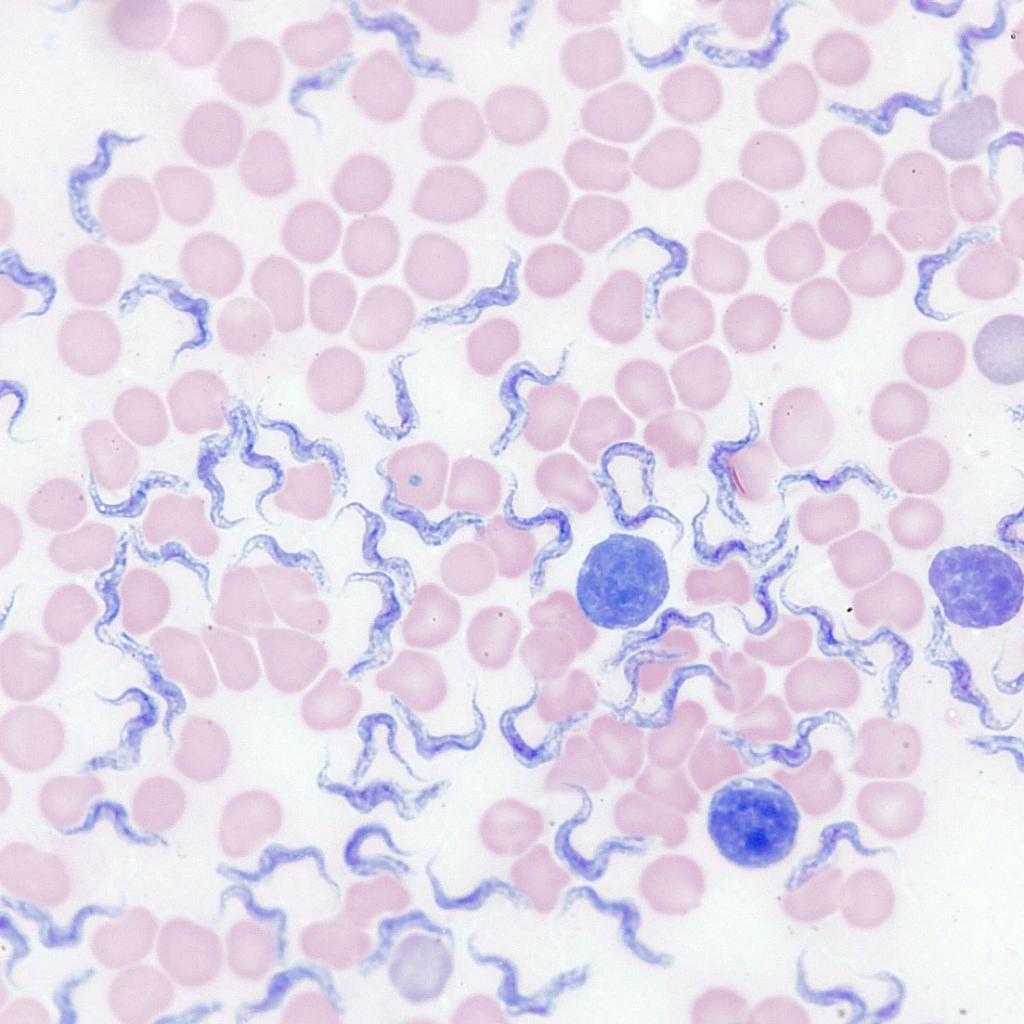This is a highly detailed microscopic image with a predominantly white background indicative of a slide, possibly dyed for clarity. Dominating the image are numerous small, distorted circular objects that are pale pink to purplish in color, likely representing cells. Interspersed among these cells are several blue squiggly lines, resembling tiny worms, adding a dynamic texture to the scene. Additionally, three larger blue circles stand out markedly; these may be about twice the size of the pink cells and are arranged roughly in a triangular formation, concentrated towards the right side of the image. These larger blue circles appear disfigured and might be potential parasites or other microorganisms, contrasting against the uniform dispersion of the smaller pink cells. The intricate interplay of colors and shapes, with blue squiggles and larger blue circles amidst a sea of pink cells, creates a complex and detailed visual that is characteristic of microscopic analysis.